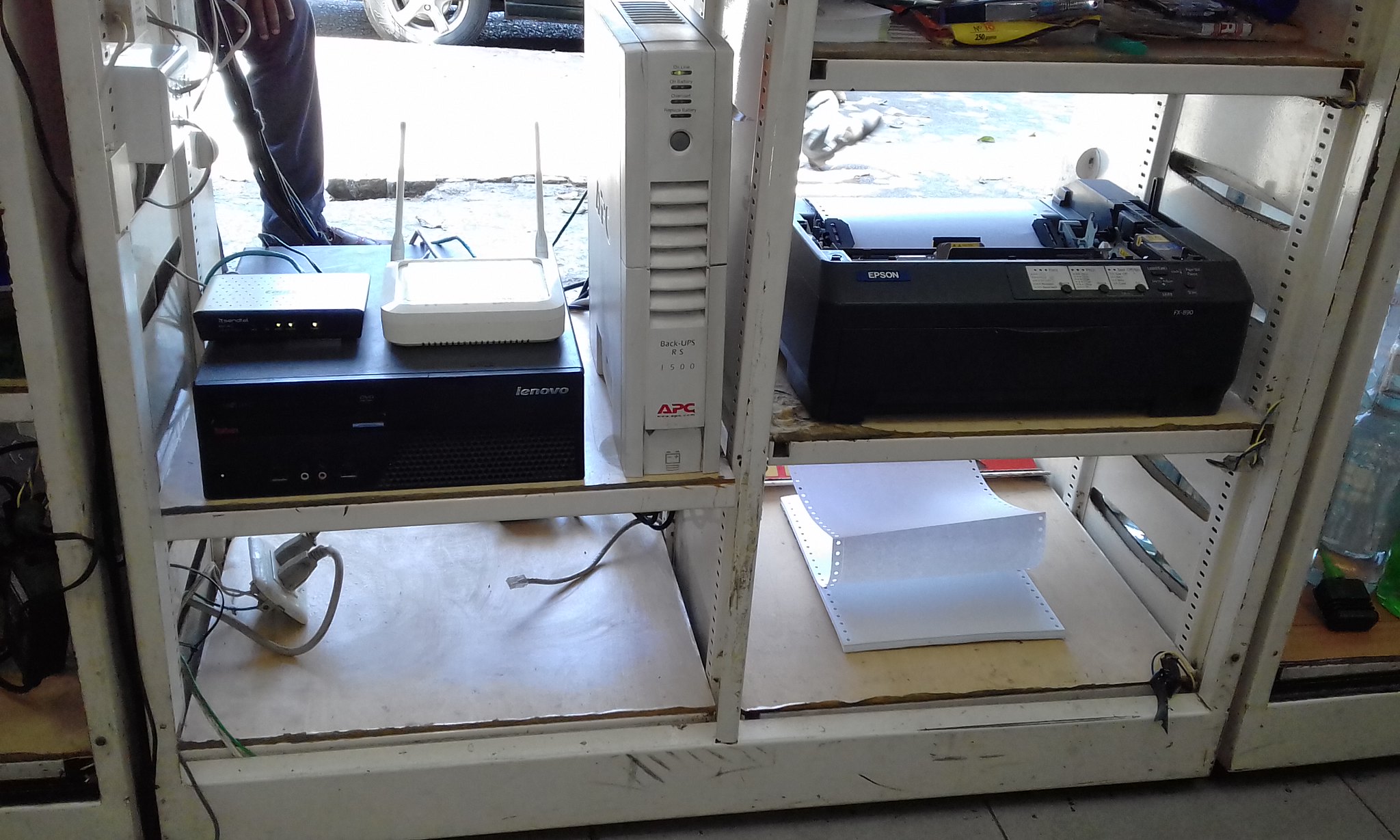This color photograph depicts a cluttered and busy setup of computer equipment on two battered white metal shelving units. The right shelving unit prominently features a black Epson printer loaded with dot matrix paper that has holes punched along the sides; the paper spills out from the printer and folds back and forth like an accordion. Below the printer is a stack of similar dot matrix paper and a tangled mess of cables plugged into a power strip, along with a dangling phone cord.

The left shelving unit holds a black box labeled "Lenovo" in the top right corner, with a router and an additional small black modem on the shelf above it. A tall white device labeled "Backups RS-1500 APC" can be seen in the background. The arrangement is set against a backdrop of adjustable shelves, and the overall scene looks disorganized, with numerous cords and miscellaneous items contributing to the chaotic feel of the image.